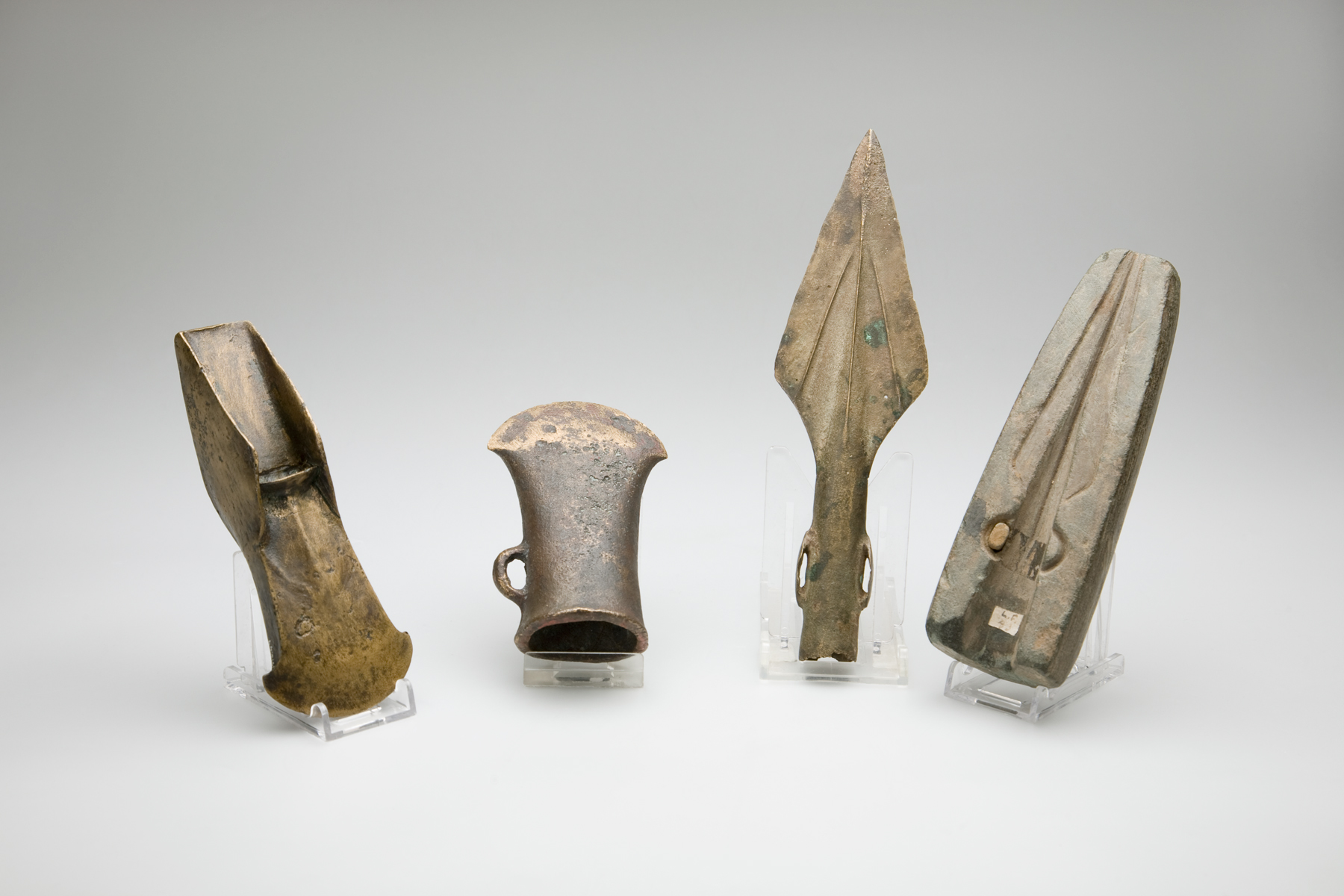The image depicts four ancient, tarnished gold or bronze-colored metal artifacts arranged side by side on clear plastic display stands against a gray background. The objects exhibit signs of aging with hues of brown, gray, and copper. From left to right, the first artifact resembles an angular, tarnished gold whistle or possibly a shovel head with a diminutive blade on one end. The second piece appears as a small pot or cup with a miniature handle, featuring a flattened bottom, evoking the appearance of a snuffer. The third item looks like a metal arrowhead or spearhead, characterized by a design groove forming an upside-down 'V' along its top. The fourth artifact is rectangular with an indented groove down the center, reminiscent of a ceremonial sword or a bar-like object. These artifacts are methodically displayed, leaning against clear stands that give the impression of picture frames, presenting them in a slight curve for better visibility.